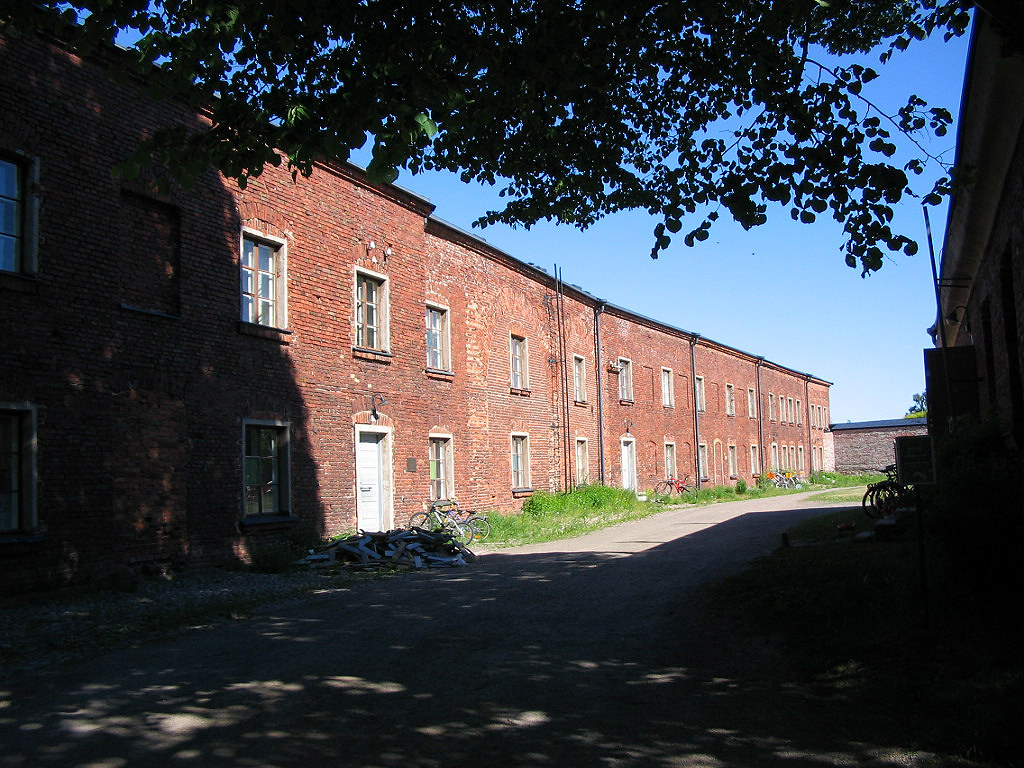This photograph captures a row of red brick townhomes, taken from a slightly diagonal angle that adds a sense of depth and perspective to the image. Each two-story townhome features seven windows—three on the left side and four on the right—with white trim around them, and white doors. In front of the closest townhome, there's an untidy stack of wooden planks and other debris, while two bicycles are parked nearby. Further down, more bicycles are stationed near the entrances of the other townhomes. The area in front of the buildings is a blend of overgrown grass and pavement, with a tan pathway or roadway that is partially obscured by shadows, making it hard to distinguish if it’s cement, asphalt, or dirt. Tree cover overhead casts substantial shadows on the left of the image and on the ground in the foreground, creating a stark contrast with the clear blue, cloudless sky above. A fire escape ladder is mounted at the center of the buildings, and trees and shrubs are visible both at the top of the photo and around the edges, their leaves appearing green where hit by the light, but mostly black due to the heavy shadowing. There is no text or wording visible in the photo. The image appears to have been taken during the daytime, as suggested by the natural lighting and shadows.